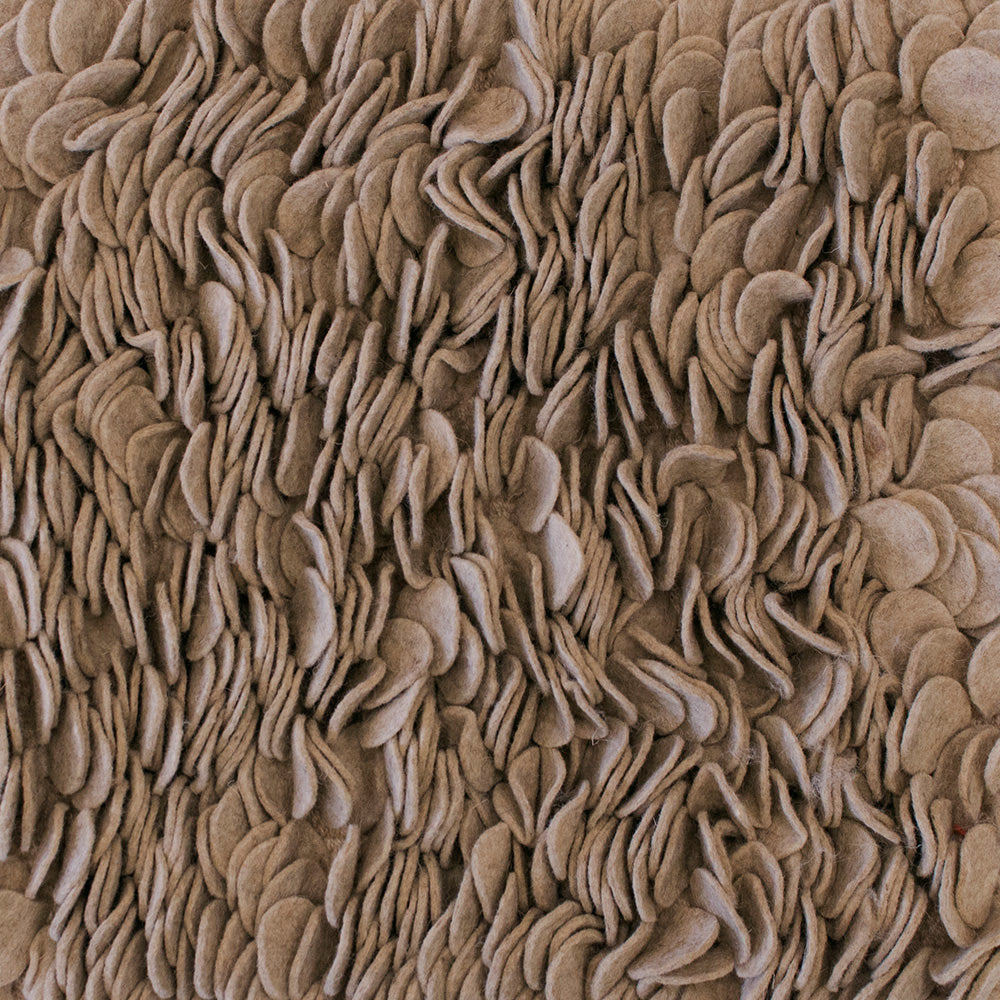In this detailed photograph, the entire frame is occupied by numerous objects that resemble thick, tan-colored chips. Their texture appears soft, potentially akin to a wool or felt material, and they have a whitish-brown, golden hue. These chips boast a rounded shape, akin to potato chips, with some displaying a slight bend. Most of the image shows their sides, giving an impression of their thickness and irregular stacking. The objects come across as felt pieces, possibly used under chair legs, rather than food items, given their uniform size and shape but haphazard arrangement. Their varying forms—some straight, others wavy—suggest a natural, unorganized pile.